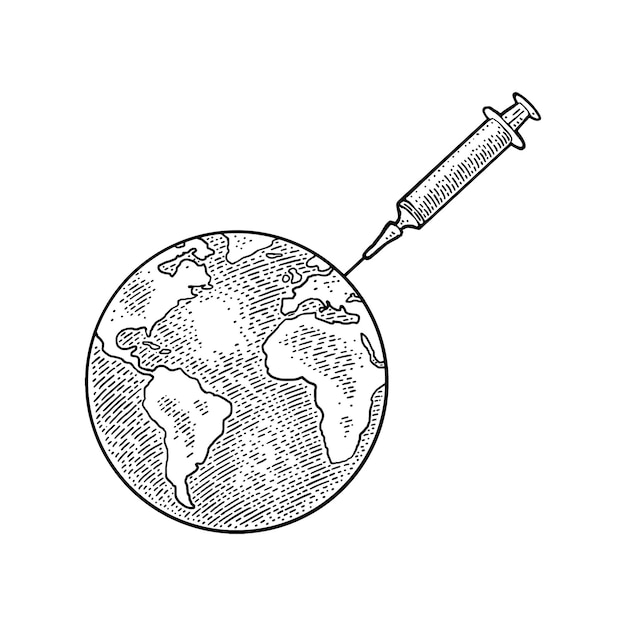This is a monochromatic, AI-generated painting featuring a stark, black-and-white color scheme. The central focus of the image is a detailed depiction of the Earth, with continents such as North America, South America, and Africa prominently displayed amidst vast oceanic expanses. A large syringe, or needle, is illustrated as being injected into the globe, symbolizing a significant, possibly ominous action being taken against the planet. The background of the painting is entirely blank, pure white, which enhances the stark and somber tone of the artwork. The absence of text and additional elements results in a minimalist yet impactful composition.